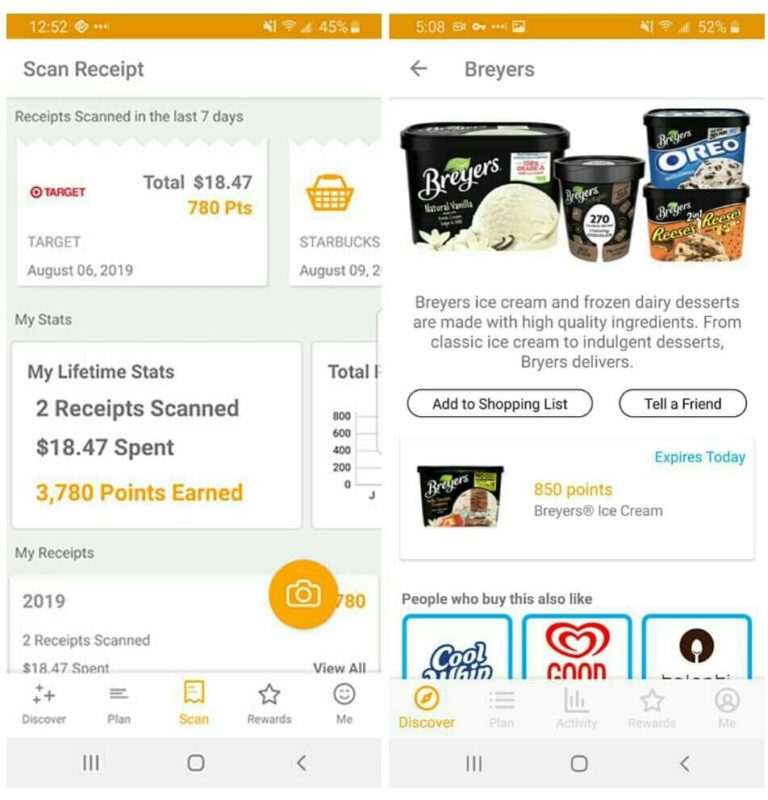Here is a detailed and cleaned-up caption for the provided image:

---

The image consists of two smartphone screenshots placed side by side, each displaying different sections of a receipt scanning app.

**Screenshot on the Left:**
- **Top Bar:** Features an orange-tinted bar showing the time as 12:52 PM and a battery life of 45%.
- **Main Section:**
  - **Header:** The text "Scan Receipt" indicates the current activity within the app.
  - **Receipts List:** Shows a categorized list of scanned receipts from the last seven days.
    - **First Receipt:** 
      - Retailer: Target
      - Date: August 6, 2019
      - Total Amount: $18.47
      - Points Earned: 780 points
      - The receipt image has a zigzag top edge, simulating a printout torn from a printer.
    - **Second Receipt:**
      - Retailer: Starbucks
      - Date: August 9, 2019
      - The right side of this receipt is partially cut off, requiring scrolling to view in full.
  - **Stats Section:**
    - **Header:** "My Stats"
    - Description: Detailed lifetime stats
      - Receipts Scanned: 2
      - Total Amount Spent: $18.47
      - Points Earned: 3,780 points
  - **Function Buttons:** Text options such as "My Receipts," "More Details," and an orange circle with a white camera icon, allowing users to take and upload photos of receipts.
  - **Bottom Navigation Menu:**
    - Options Available: Discover, Plan, Scan, Rewards, and Me
    - The "Scan" option is currently highlighted in orange, indicating the active section, while the others are in blue.

**Screenshot on the Right:**
- **Top Bar:** Displays an orange-tinted bar with the time as 5:08 PM and a battery life of 52%.
- **Main Section:**
  - **Advertisement Section:** Prominently features a Breyers ice cream promotion.
    - **Image Display:** Includes photos of various Breyers ice cream products:
      - Flavors/Types: Vanilla ice cream, a possible low-carb option, and stacked Oreo and Reese's Pieces flavored ice cream.
    - **Description:** "Breyers ice cream and frozen dairy desserts are made with high-quality ingredients. From classic ice cream to indulgent desserts, Breyers delivers."
    - **Action Buttons:** Two blue-outlined buttons for user interaction:
      - "Add to Shopping List"
      - "Tell a Friend"
    - **Offer Details:** Notation that the offer expires today, providing 850 points for buying Breyers ice cream.
  - **Related Products Section:** Displays suggested items with three blue squares indicating popular choices such as Cool Whip, Good Humor products, and Talenti frozen treats.

Overall, the screenshots provide an insightful look into a receipt scanning and reward-earning app, highlighting recent activities, available offers, and user engagement features.

---